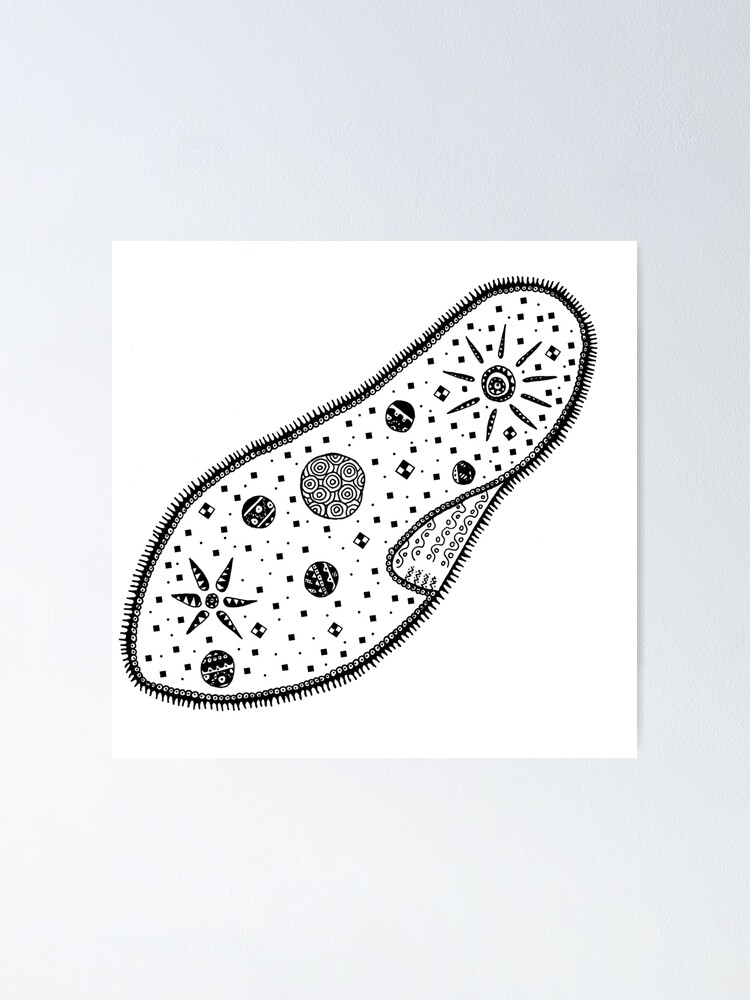The artwork presents a captivating black and white image of a foot-shaped object, centered on a white canvas square with a surrounding gray background. The foot impression is densely populated with a myriad of intricate designs: crisscrossing squiggly lines, star motifs, and celestial representations, including sun and planets. There are also numerous dots and tiny squares scattered throughout, resembling a field of minute elements. Additionally, two prominent circular areas with radiating spikes are interspersed among the designs, contributing to a celestial or cellular theme. The edges of the foot outline are punctuated with small, sharp spikes, further adding to the detailed and textured appearance. The overall effect is a mesmerizing blend of artistic complexity, suggestive of an ink or digitized medium, with no accompanying text or labels.